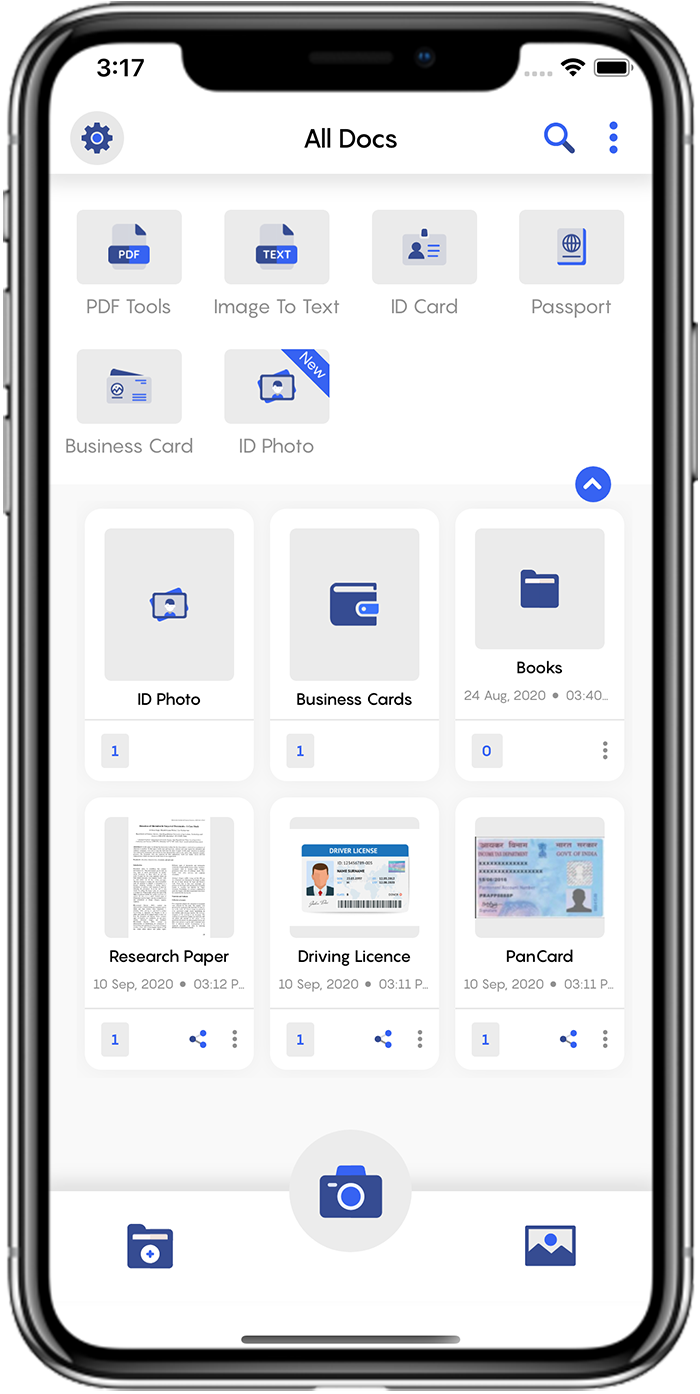The image portrays a smartphone with a clearly visible outline, displaying various functional details. On the right side of the device, the power button and volume controls are discernible. The phone screen is active, showing the current time of 3:17 PM. The top-right corner of the display includes icons indicating WiFi connectivity and battery status. 

Centrally positioned beneath the time is the label "All Docs," flanked by a magnifying glass icon for search functions, a three-dot menu for settings on the right, and a gear icon on the left for additional settings.

Below this header, four distinct icons are arranged horizontally. The first is a PDF file icon, followed by an "Image to Text" icon, an ID card icon, and a passport icon. Further down, two more icons are displayed: one representing a business card and another an ID photo, the latter being a new feature.

Moving further down, there are three boxes showing uploaded items: 
1. A photo ID with the count of 1.
2. A business card, also with the count of 1.
3. A book with a count of 0.

Additionally, the screen shows a research paper uploaded on August 24, 2020, with the designation "312," the meaning of which is unclear. Another entry is a driver's license with a more colorful and detailed clip art, uploaded on September 10, 2020, also showing a count of 1.

Each entry provides its uploaded date and time, the quantity of uploads, and options for sharing and settings. There is also functionality for users to add new files via a plus button, view existing photos, or directly capture new images using the camera button; the latter being centrally and lower positioned on the screen.